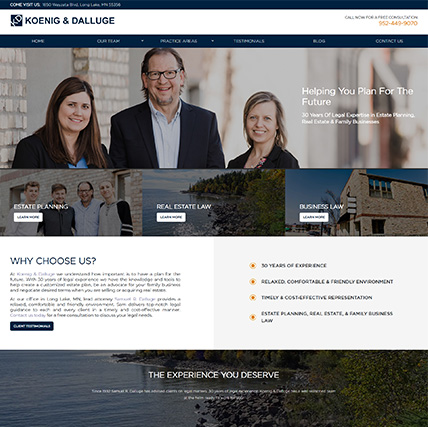The home page of the Koenig & DeLuge website, a law firm specializing in real estate planning and family businesses, is designed to welcome visitors with an invitation to "Come visit us." The site features a navigation menu with categories such as Home, Blog, Contact Us, and Testimonials. Although some menu items are slightly blurry, their purposes are discernible. The main image showcases three smiling individuals: a female with long brown hair in a black coat over a blue shirt, a taller gentleman with short brown hair, glasses, and a goatee in a black coat with a blue undershirt, and another lady with dirty blonde hair also dressed in a black coat. Adjacent to the photograph is the firm's motto: "Helping you plan for the future," highlighting their 30-year expertise. Below the image are accessible buttons for Real Estate Law, Business Law, and Estate Planning.